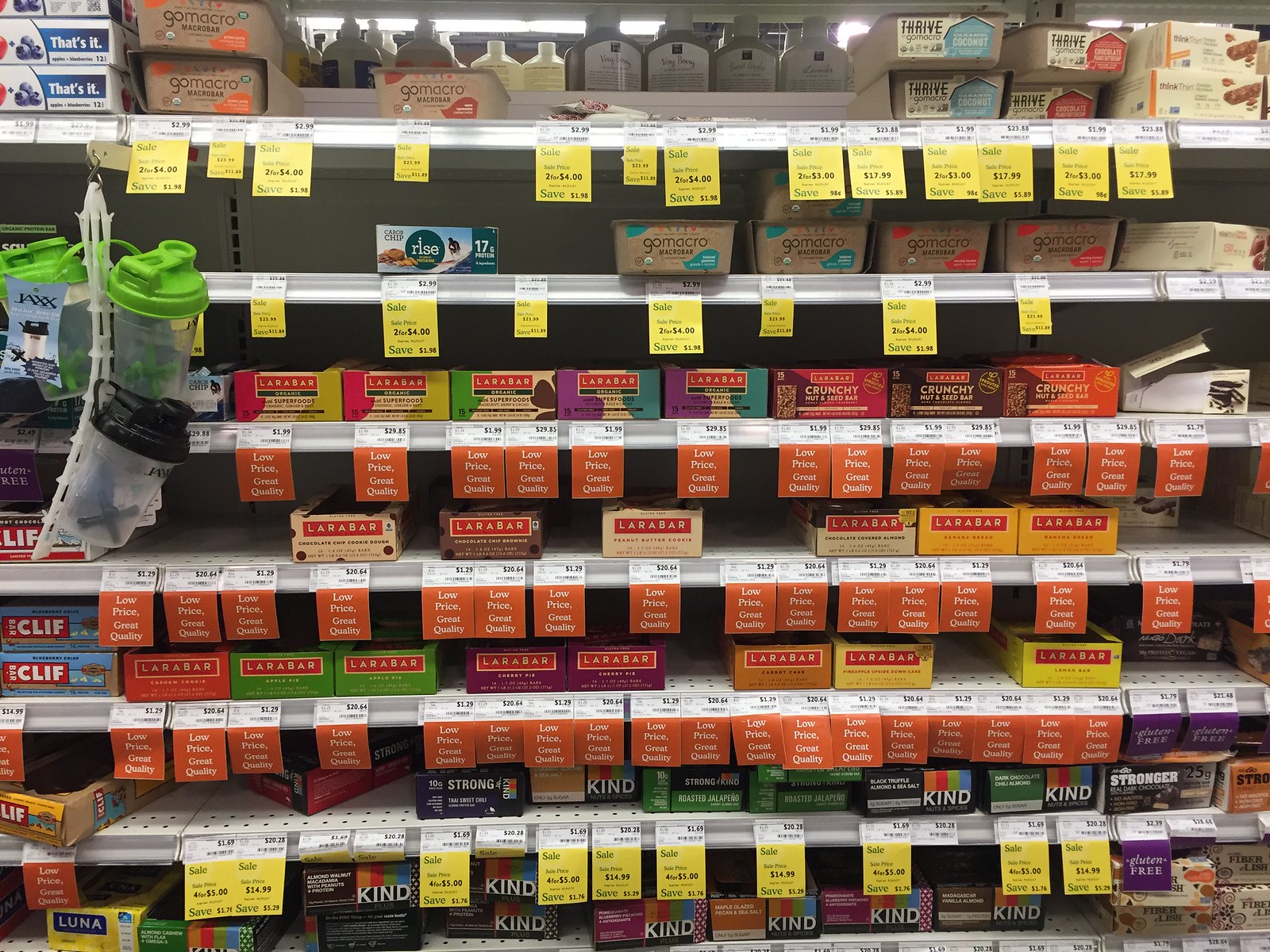A well-stocked grocery store shelf filled with a wide variety of energy bars, including popular brands like Kind, Lara Bar, Clif Bar, and Luna. Each shelf showcases multiple flavors from these brands, making for a colorful and organized display. Several yellow sale tags are prominently featured, drawing attention to the discounted prices. In the background, on the opposite side of the aisle, there are bottles visible on adjacent shelves. Additionally, there is a hanging display of protein shaker cups, equipped with agitators for efficient mixing.